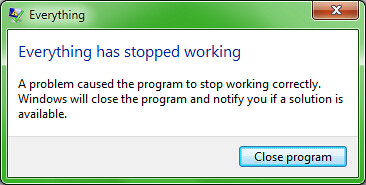The image depicts a rectangular application window on a computer screen, bordered by a bright green-colored frame that is narrow along the bottom and sides but thicker at the top. In the top left corner, next to a small computer icon, the title reads "everything" in black font. In the top right corner, there is a small, glossy red rectangle with curved corners and a white X in the middle, symbolizing the close button. Inside the window, set against a light gray background, blue text states "everything has stopped working," followed by red text indicating, "a problem caused the program to stop working correctly. Windows will close the program and notify you if a solution is available." At the bottom right, within a gray bar, there is a light blue button with black text that reads "close program." The overall design and elements resemble a typical error dialogue box from Windows Vista or Windows 7.